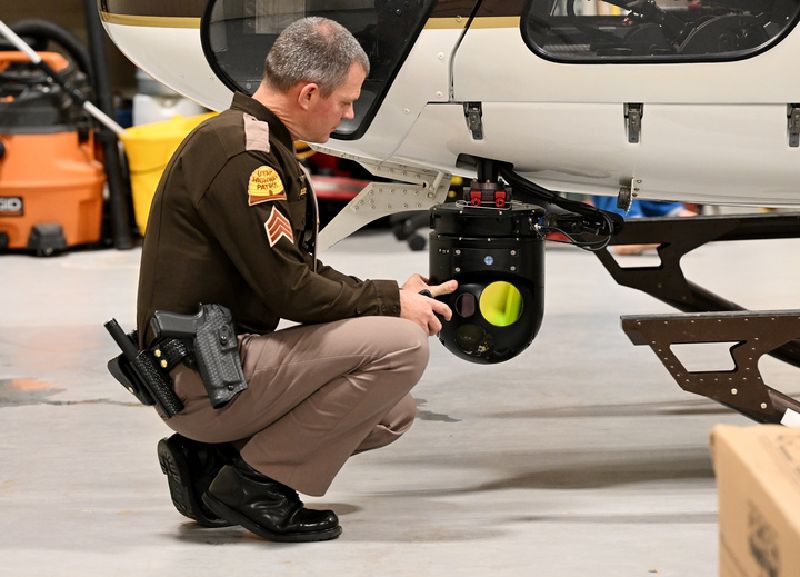The color photograph features a man in a police or sheriff uniform, consisting of shiny black shoes, khaki pants, and a dark brown, long-sleeve button-up shirt adorned with various patches. One patch on his sleeve features a three or four-striped design, and another resembles a beehive or stars and bars insignia. The man, profiled sideways to the camera, is squatting down and meticulously adjusting a camera attached to the bottom of a helicopter. Strapped to his side is a pistol, part of a utility belt equipped with various police tools. In the background, tools and a shop vacuum are visible, suggesting the setting is a maintenance or workshop area.